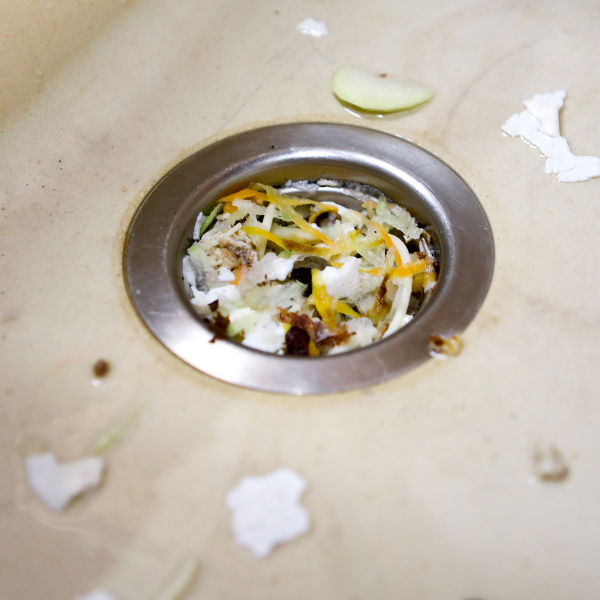This image is a close-up view of a kitchen sink's drain, which is silver in color. The surrounding sink has a white, marbly finish with some brown aging or discoloration spots. The drain is clogged with various food items, including pieces of vegetables such as orange, yellow, and white segments, green cucumbers, thin apple slices, and possibly some coconut flakes or thin orange slices. Additionally, there are some pieces of tissue paper and even elements resembling lettuce or salad. Water is pooling around the clogged drain, unable to pass through due to the blockage, and there are a few brown spots scattered throughout the sink's surface.